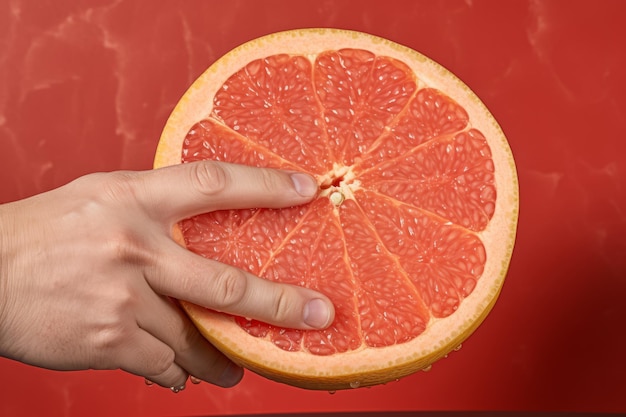The image depicts a freshly sliced half grapefruit positioned against a striking background filled with various shades of orange and red, interspersed with white streaks that create a marbled effect. A person's right hand is prominently placed on the fruit, with two fingers extended in a distinctive pose: one finger is touching the center of the grapefruit while the other is placed towards the edge, showing the impressive size of the fruit, almost comparable to a melon. The grapefruit's outer skin showcases a yellow hue, while the juicy interior reveals the characteristic pinkish-red flesh divided into neatly arranged sections that resemble slices of pie. This unique hand placement suggests a potential measurement or simply an emphasis on the fruit's size and freshness.